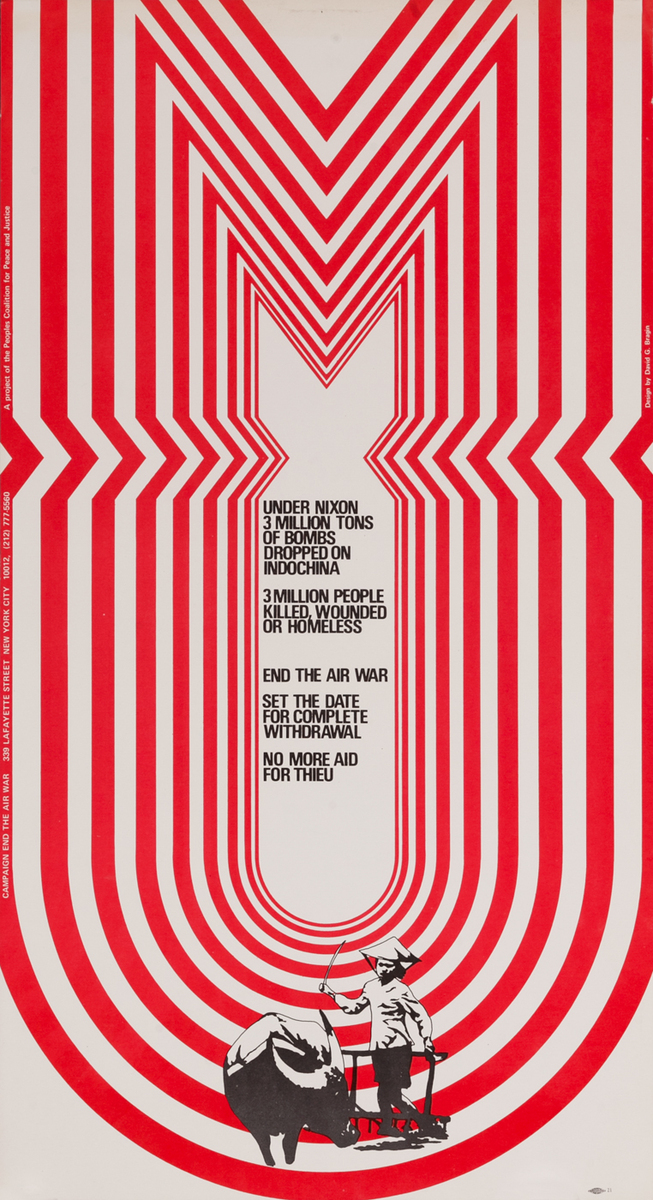This is a vertically rectangular, borderless poster with an off-white background. Dominating the center of the image is an old-fashioned World War II-era bomb design, constructed from alternating red and white lines that create a visually striking, repeated pattern. The bomb shape, abstract yet recognizable, houses a poignant message: "Under Nixon, 3 million tons of bombs dropped on Indochina. 3 million people killed, wounded, or homeless. End the air war. Set the date for complete withdrawal. No more aid for THIEU." Below this stark message, a pencil drawing captures a poignant scene of a Vietnamese farmer in Southeast Asia, riding a plow drawn by an ox, providing a sharp contrast to the destructive imagery above. The overall design emphasizes the devastating human impact of the air war in Indochina during Nixon's presidency.